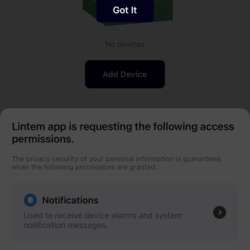Screenshot of a heavily compressed and low-quality image featuring a grayed-out interface. A semi-transparent black gradient overlays the image, obscuring details. At the top, a button labeled "Got it" is visible, followed by another button that says "Add a Device." The text "Lintam app is requesting the following access permissions" is partially discernible but appears intentionally blurred. Additional notifications follow below, but the text remains indecipherable due to blurriness and heavy compression artifacts. The image resolution is significantly reduced, making it difficult to read or understand. Overall, the image quality is poor and seems to have been resized, contributing to its lack of clarity and detail.